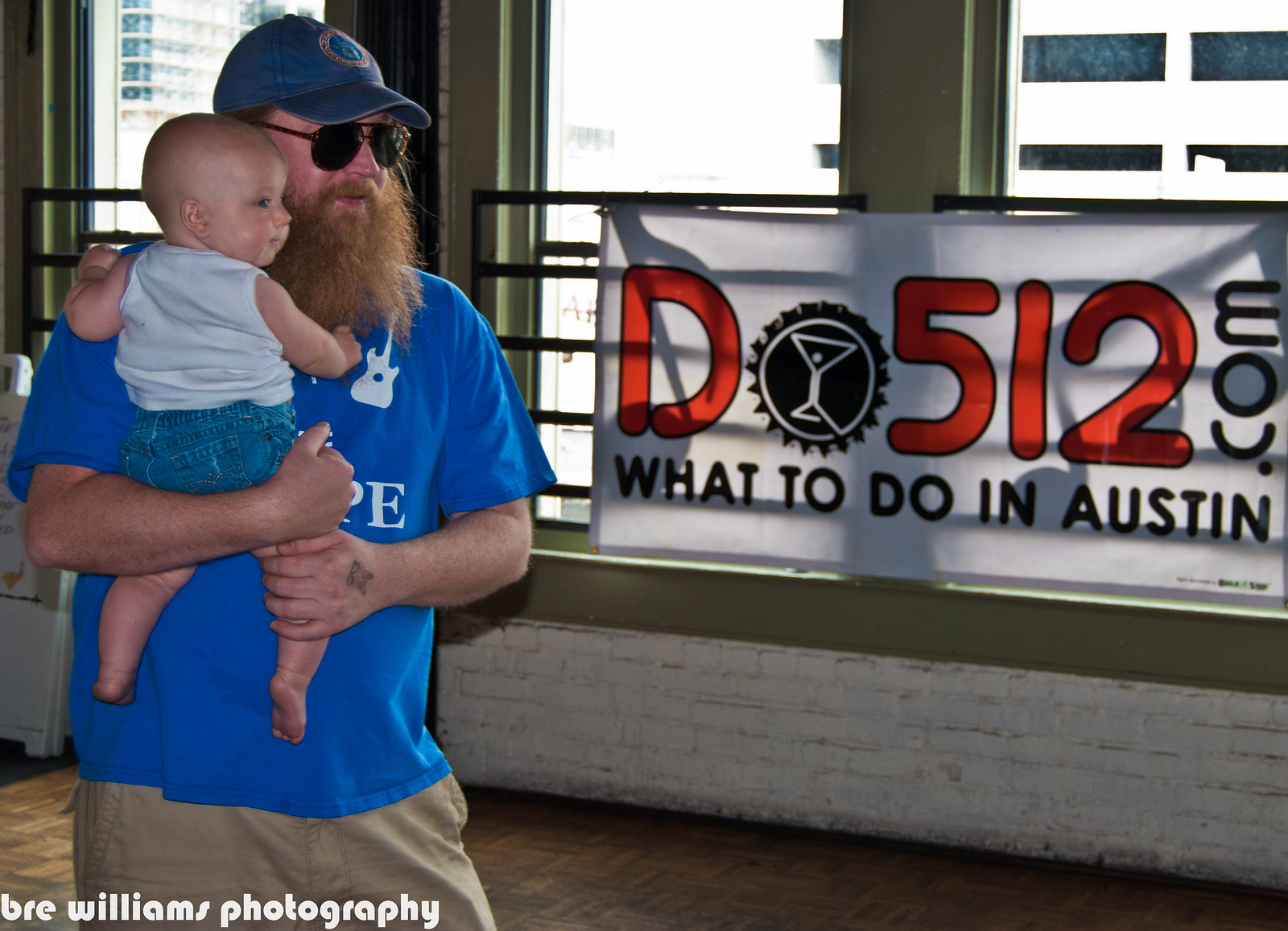In this photograph, on the left side, there is a man with a notable, long red beard, wearing a blue baseball cap featuring a circular blue and red emblem on the front, and red-framed aviator sunglasses. He is dressed in a short-sleeved blue t-shirt adorned with a white guitar design and some indistinct white lettering, paired with beige pants. Nestled in his right arm is a young baby, probably under a year old, dressed in a white tank top and blue jean shorts. Both the man and the baby appear to be looking slightly off to the right. In the background, there are three large windows with green frames set into a brick wall, and a wooden lattice flooring is visible below. Draped in front of the windows is a white banner with black text that reads "DO512.com, what to do in Austin."